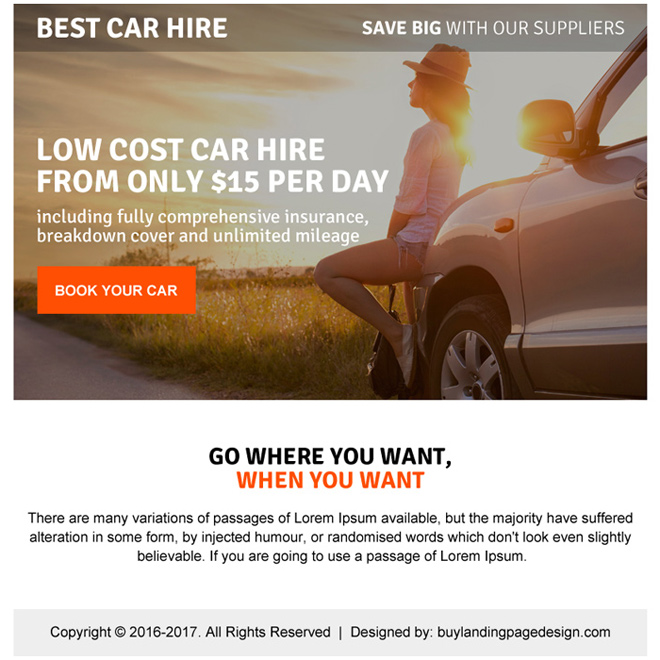The image is a promotional screenshot for a car hire service. At the top left corner, in bold white capital letters, it reads "BEST CAR HIRE," while to the right, it states "Save Big with Our Suppliers." Below this, there is a photograph showcasing only the front driver's side of a car with a woman sitting on its hood. The woman is dressed in very short shorts, revealing her left leg, and she is wearing a white shirt that reaches her elbows and a hat resembling a fedora. Due to the silhouette effect, her face is not clearly visible. The backdrop suggests a serene sunrise or sunset, as indicated by the rays of the sun visible between her and the side mirror. On the left side of the image, golden fields, possibly of crops, stretch out into the distance.

Prominent in the center, a headline proclaims "LOW-COST CAR HIRE FROM ONLY $15 PER DAY" in bold, white capital letters. Below this, additional text outlines the benefits: "Including fully comprehensive insurance, breakdown cover, and unlimited mileage." An orange rectangle beneath this text features the call-to-action "Book Your Car" in white letters.

Further down, against a white background, black text reads "Go wherever you want" followed by orange text stating "when you want." At the very bottom, enclosed within a gray border, it states, "Copyright 2016 to 2017 All rights reserved," with the note "Design by landingpagedesign.com."